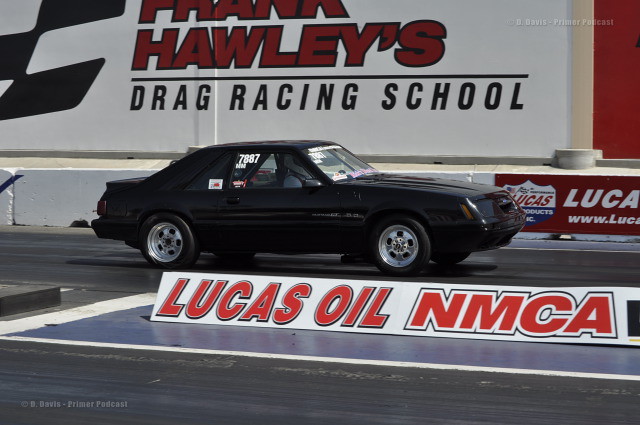The image captures a black, two-door hardtop Ford Mustang elaborately modified for drag racing. The vehicle boasts silver alloy wheels and is adorned with numerous racing decals, including the number 7887 prominently displayed on its windshield and passenger side. The Mustang is stationary and positioned at the entrance to a drag strip, just over the starting line.

In the foreground, there is a sign reading "Lucas Oil" and "NMCA," framed in red and black, and additional advertisements for Lucas Oil and "Holley's Drag Racing School" are highly visible on a large white wall in the background. A cement barrier runs behind the car, further emphasizing the racing context.

Inside the vehicle, a driver is strapped in, his safety harness secured, and he is wearing a white racing helmet. The photograph itself is a rectangular shot, wider than it is tall, and bears watermarks on the upper right and lower left corners that state "D. Davis Premiere Podcast."